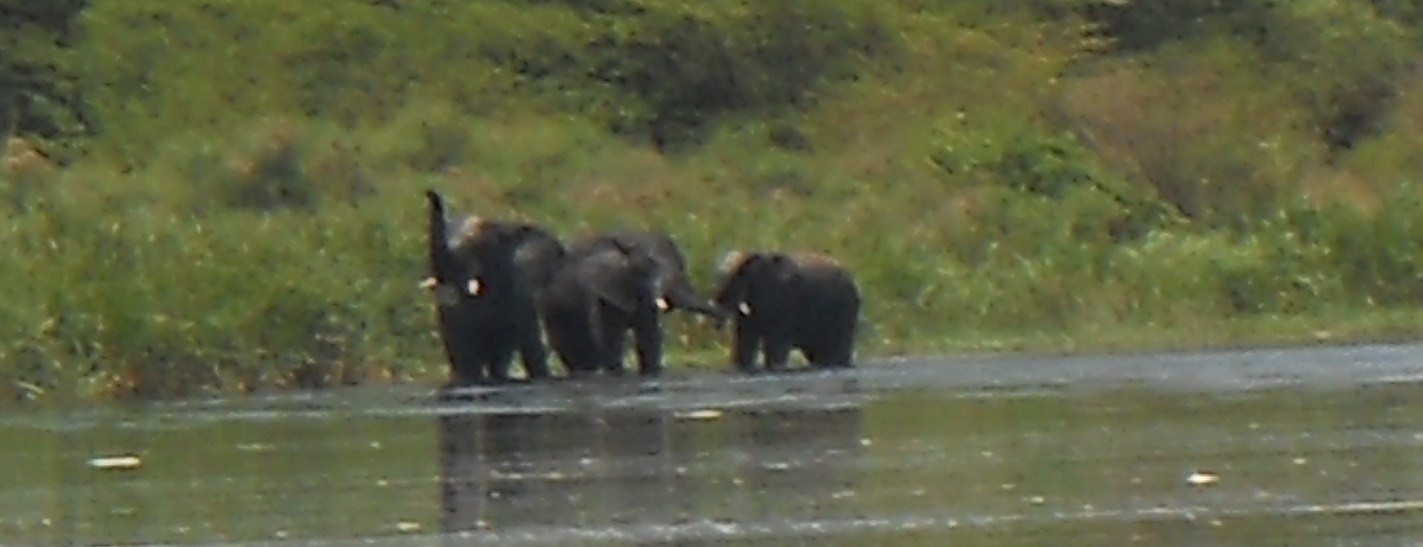This wide-angle, distant shot captures three small elephants bathing in a dark, murky river. The photo is very grainy due to the extreme zoom. The scene is set in a completely green space, featuring a lush hillside blanketed with very tall grass and bushes, stretching across one third to two-thirds of the way down the picture from right to left. The river’s shoreline, with scattered leaves floating on the water, runs across the lower portion of the image. The elephants, knee-deep in the water and appearing black due to the distance, are slightly blurry and out of focus. 

The three elephants display distinct postures: the one on the left has its trunk triumphantly raised high in the air and displays its white tusks prominently. The middle elephant faces the right, partially turned towards the left, with its head slightly tilted, showing the side of its gray body, part of its trunks, and both tusks. The elephant on the right, also gray with visible white tusks and part of its trunk, is primarily facing the left. The backdrop of tall, lush greenery adds a vibrant contrast to the scene, highlighting the wild, natural environment.